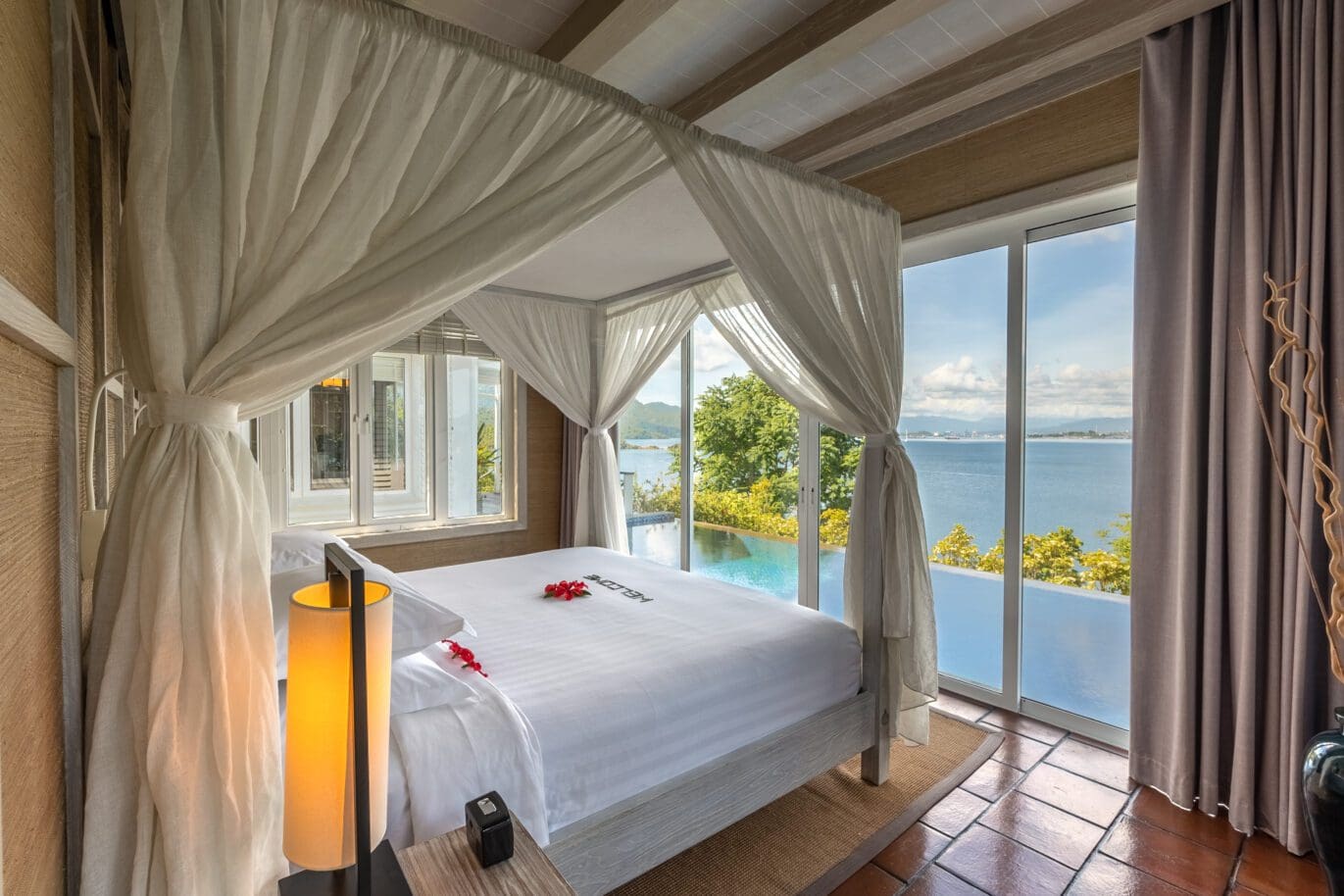This detailed photograph captures the interior of a luxurious hotel bedroom looking outward through a glass wall towards a stunning view. The room features a grand, canopy-style bed adorned with super white sheets and light gray accents, creating a serene and inviting atmosphere. The bed's gray-painted wooden frame supports white curtains that hang delicately from its corners, enhancing the elegance of the space. Positioned near the bed is a lit lamp, casting a warm glow on the room's large square brown tile flooring, which is complemented by a tan-colored rug beneath the bed. The ceiling, painted white with prominent tan support beams running horizontally, adds to the room's architectural charm. The flooring features a clay-like orange hue that harmonizes with the room's overall aesthetic. 

The focal point of the photograph is the expansive glass wall at the foot of the bed, featuring two sliding doors with large gray curtains pulled to one side. This glass barrier not only invites natural light into the room but also frames the breathtaking outdoor scene. Just beyond the room's threshold lies an infinity pool, seamlessly connecting to a landscape dotted with trees and extending toward a vast body of water—an ocean or a sea—that stretches to the horizon. This impeccable blend of indoor comfort and outdoor splendor creates a tranquil and picturesque retreat.